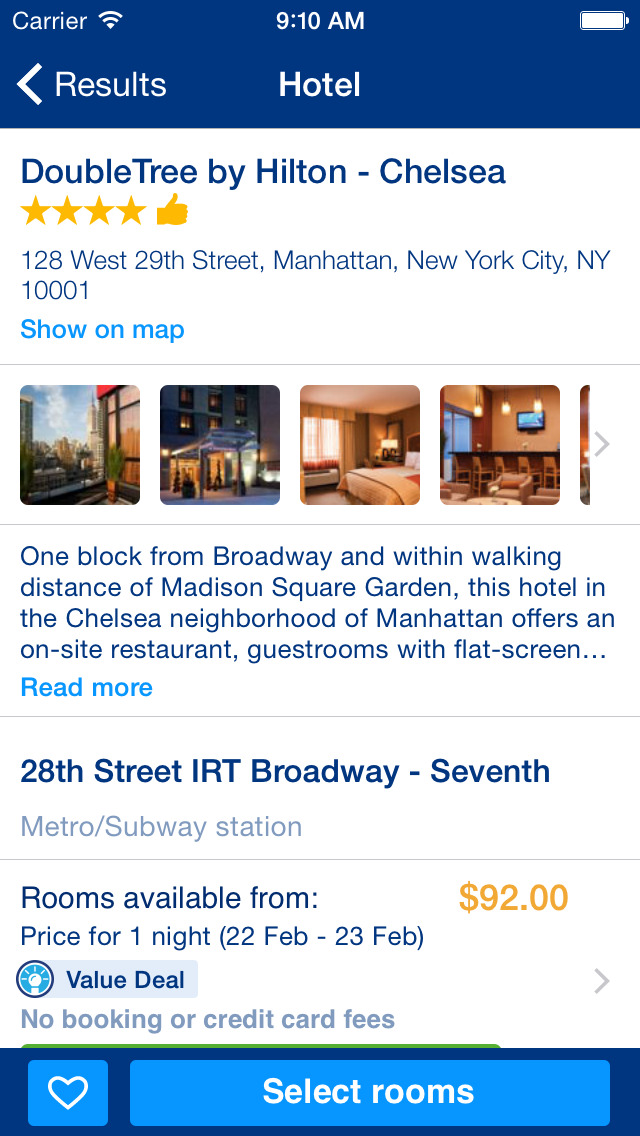A mobile phone screen displaying a travel booking site, focused on hotel reservations, is shown in the image. The screen's interface includes essential information at the top: carrier signal, full Wi-Fi bars, the time at 9:10 a.m., and a fully charged battery indicator. A blue header features the back arrow labeled 'results' and 'hotel' in the center.

The DoubleTree by Hilton in Chelsea is prominently listed in blue text beneath the header, marked with four guitar icons and a thumbs-up symbol. The hotel’s address is displayed: 128 West 29th Street, Manhattan, New York, 10001, with an interactive "show on map" link in blue. Accompanying the listing are four images showcasing different areas of the hotel: a balcony, a street view, the front entrance, a bedroom, and a room that could be either a conference area or a restaurant.

A description highlights the hotel’s prime location, one block from Broadway and within walking distance of Madison Square Garden, situated in the Chelsea neighborhood of Manhattan. The hotel offers an on-site restaurant and guest rooms equipped with flat-screen TVs. A "read more" link in blue text invites further exploration of amenities.

Additional details include the nearby 28th Street IRT Broadway and 7th Avenue subway station and room rates starting from $92 per night for specified dates (February 22 to February 23). A beacon icon denotes a "Value Deal," emphasizing no booking or credit card fees. At the bottom, a blue bar features a white heart in a light blue square (likely a favorite icon) on the left, and a light blue "select rooms" button on the right.